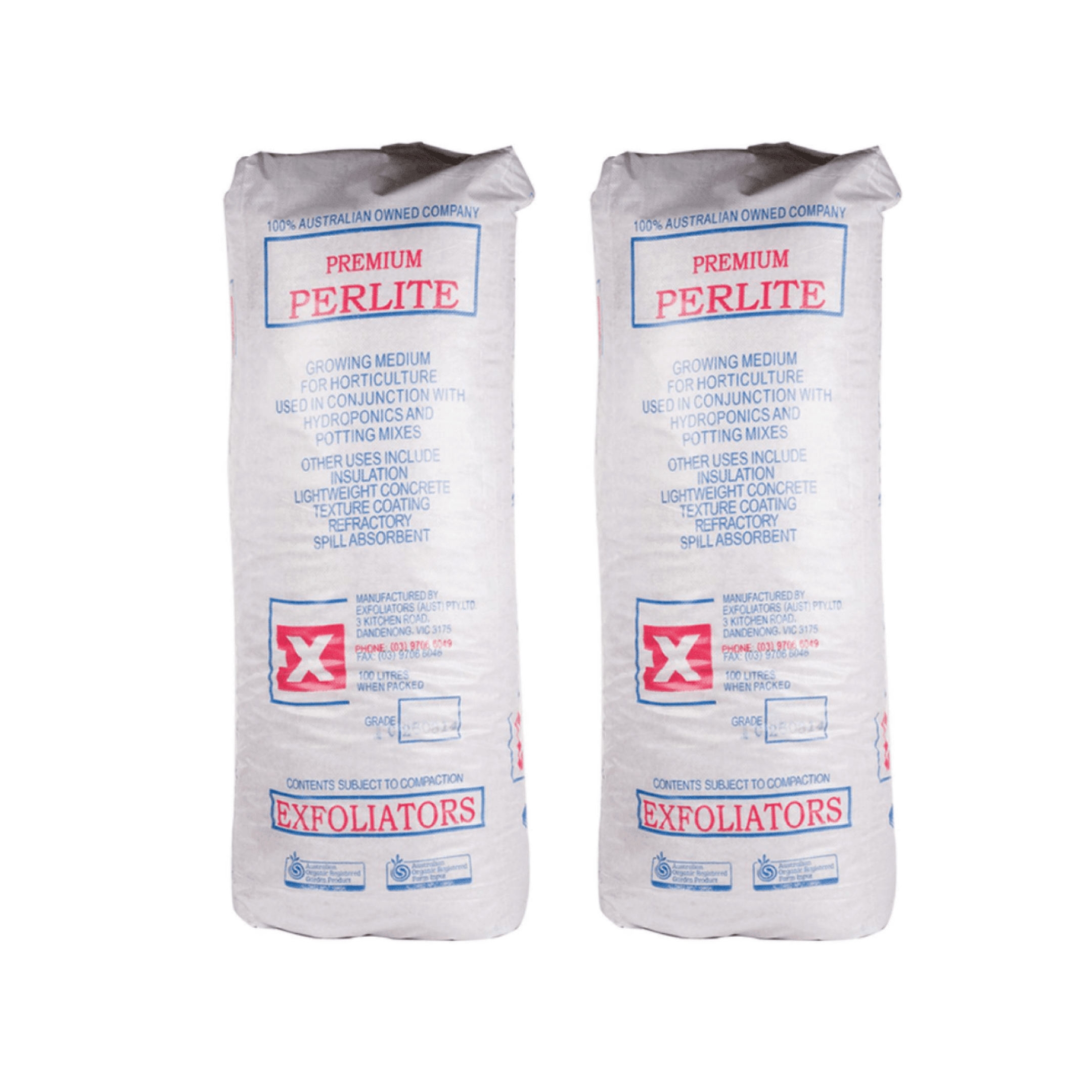The image features two identical white rectangular packets displayed side by side against a completely white background. The top of each packet reads "100% Australian owned company" in bold print. Below this, a prominent blue rectangle contains the red text "Premium Perlite." The packets describe the product further, indicating it is a "growing medium for horticulture," useful in conjunction with hydroponics and potting mixes. Additional applications listed include "insulation, lightweight concrete texture coating, and refractory spill absorbent." Near the bottom, details about the manufacturer, "Exfoliators," are provided, along with a reference to the packaging capacity of "100 liters when packed." Smaller font information and a red box with a white "X" are also visible at the bottom of the packet.